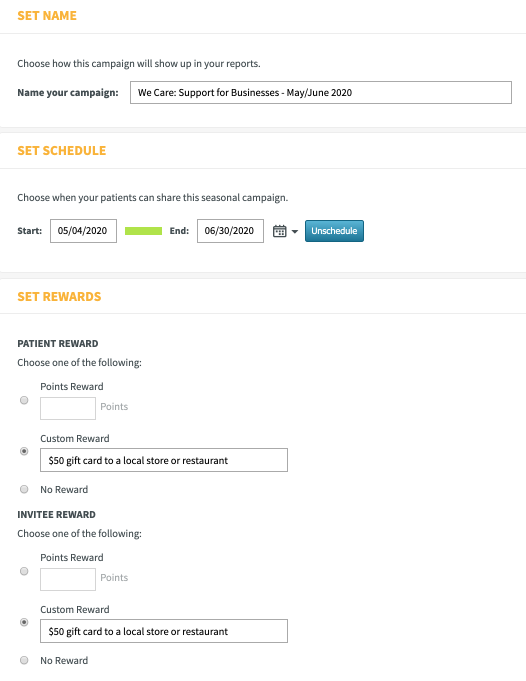Screenshot showing campaign setup options with various customization features. The interface includes fields such as "Set Name" which allows the user to choose how the campaign will appear in their reports, with a suggested campaign name "We Care - Support for Business, May-June 2020". 

In the "Set Schedule" section, users can select the timeframe for the campaign, indicating it starts on May 4, 2020, and ends on June 30, 2020. This section specifies that users can decide when patients will be able to share the seasonal campaign.

The "Patient Reward" section offers a choice among different reward options: 
- Points Reward
- Custom Reward
- $50 Gift Card to a Local Store or Restaurant
- No Reward

Similarly, the "Invitee Reward" section provides the same reward options, indicating that a $50 gift card has already been selected. Within both reward sections, the "No Reward" and "Points Reward" options are displayed in gray text, while the other selectable options are in bold black text.

Highlighted in orange are the key setup steps "Set Name," "Set Schedule," and "Set Rewards," guiding the user through the campaign creation process. The screenshot also features a blue box behind an unspecified "unscheduled" action. The purpose of this blue box remains unclear as it is repeated without additional context.